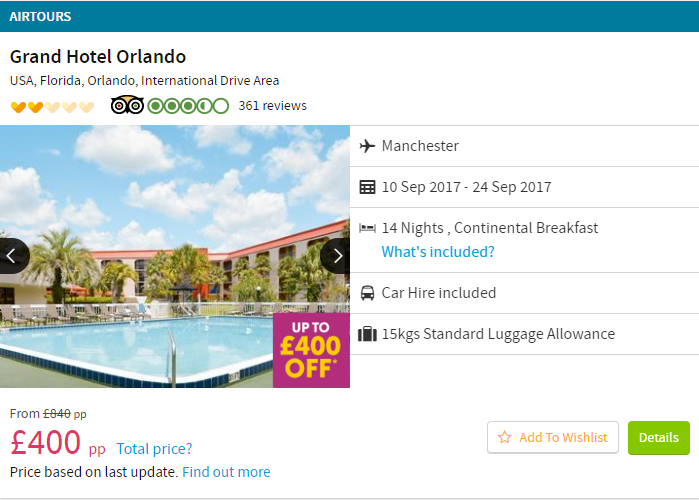The image features a promotional banner for air tours in the Orlando, Florida area. The top section displays "Air Tours" in white font on a blue horizontal bar, which spans from left to right. Below this, the image background is white, contrasting with the prominent black text that reads "Grand Hotel Orlando". Underneath, a smaller text specifies the location as "USA, Florida, Orlando, International Drive area".

Further down on the left side, a rating system is depicted with five heart icons, two of which are filled in. Adjacent to this, there is a logo resembling owl eyes, indicating a score with three and a quarter filled in circles, based on 361 reviews.

At the very bottom, the text states that the departure airport is Manchester, with travel dates from the 10th to the 24th of September 2017.